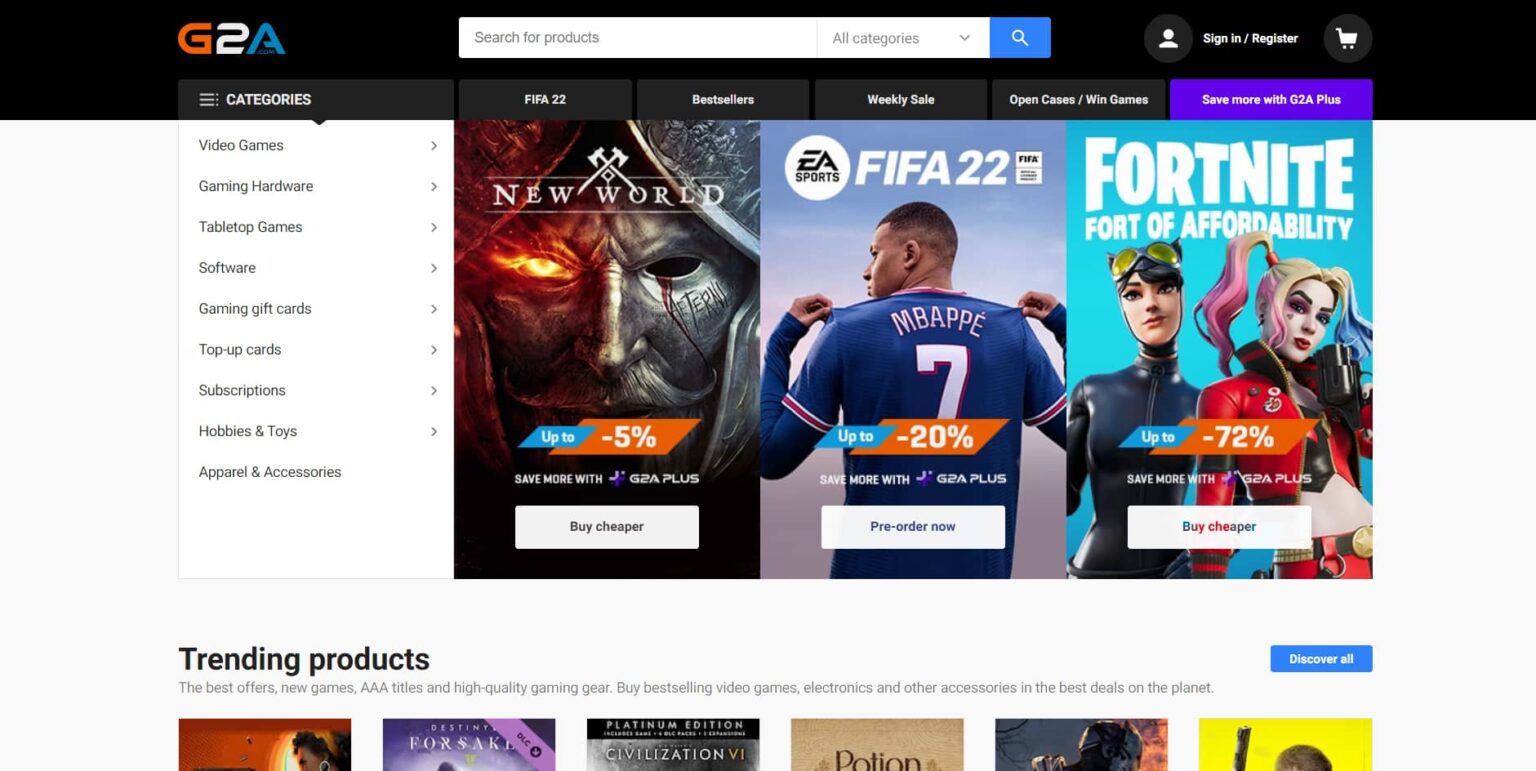The image shows the interface of a website, prominently featuring the G2A logo, with the letter "G" in orange, the number "2" in white, and the letter "A" in blue. At the top of the page, there is a search bar with a blue magnifying glass icon and options labeled "Search for products" and "All categories." The main section of the page showcases several video games available for purchase. Titles like "New World," which features an image of a mask, "FIFA 22," and "Fortnite: Fort of Affordability" are displayed, each adorned with discount badges indicating savings percentages (e.g., up to -5%, -20%, and -72%).

The games are promoted with the message "save more with G2A+" and have white buttons below them labeled either "Buy Cheaper" or "Pre-order Now" depending on their release status. The bottom section of the page teases additional games listed under "Trending Products," with related categories such as "The Best Offers," "New Games," "AAA Titles," and "High Quality Gaming Gear." The call-to-action button "Discover All" is in blue.

On the left sidebar, a comprehensive list of categories is displayed, including "Video Games," "Gaming Hardware," "Tabletop Games," "Software," "Gaming Gift Cards," "Top Up Cards," "Subscriptions," "Hobbies and Toys," and "Apparel and Accessories." The website promotes itself with claims like "Buy best selling video games, electronics, and other accessories with the best deals on the planet."